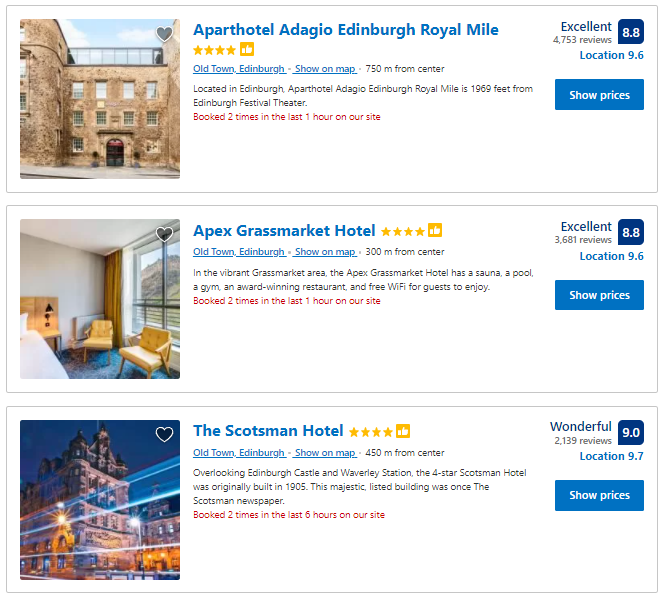The screenshot showcases a search results page for hotels, displaying three options with associated details. Each hotel listing is accompanied by a color image and relevant information.

The first listing is for the Apart Hotel Adagio Edinburgh Royal Mile. It features a star rating, clickable links for more details or bookings, and a brief description of the hotel. On the far right, there is a verbal summary of the hotel, the number of reviews, and a digital rating score.

The second listing is for the Apex Grassmarket Hotel, following the same structure as the first. It includes a description, star rating, clickable links, and a summary with the number of reviews and digital ratings.

The third listing is for the Scotsman Hotel. This hotel has the highest rating among the three, with a score of 9.0 and a description categorized as 'wonderful.' The first two hotels, Apart Hotel Adagio Edinburgh Royal Mile and Apex Grassmarket Hotel, both have ratings of 8.8, described as 'excellent.'

Each listing provides critical information to help users compare and decide on a place to stay based on descriptions, reviews, and ratings.